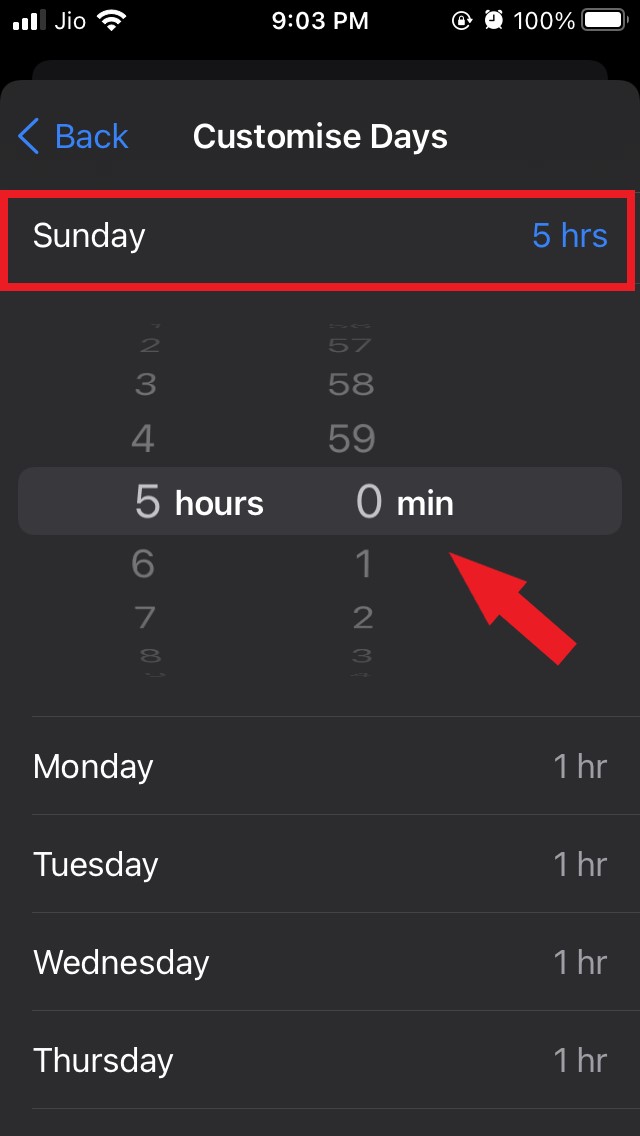The screen has a minimalist design with a black background. At the top, there is a blue arrow pointing to the left accompanied by the word "Back," also in blue. Next to that, the text "Customise Days" is displayed in white, with "Customise" spelled in the British English manner.

Below this heading is an elongated red rectangle containing the word "Sunday" in white font. To the right of "Sunday," the screen shows "5 hours" in blue text. Beneath this section, there are two columns of numbers: one column lists the hours 3, 4, 5, 6, and 7, while the other column lists the minutes 58, 59, and 0. The current selection is highlighted in bold, displaying "5 hours and 0 minutes." A red diagonal arrow ascends from the bottom and points to the selected time of "5 hours and 0 minutes."

Following the Sunday section, the screen lists:
- "Monday" in white text with "1 hour" to the right.
- "Tuesday" in white text with "1 hour" to the right.
- "Wednesday" in white text with "1 hour" to the right.
- "Thursday" in white text with "1 hour" to the right.